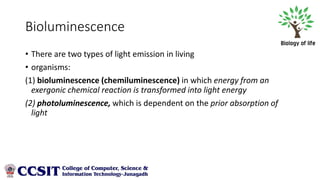The image is a slide from a PowerPoint presentation, predominantly white with black text. The title at the top reads "Bioluminescence" and is situated to the right side. Below the title, there are two bullet points explaining the types of light emissions in living organisms. The first bullet point describes "Bioluminescence (Chemiluminescence)," noting that energy from an exergonic chemical reaction is transformed into light energy. The second bullet point outlines "Photoluminescence," which depends on the prior absorption of light.

In the top right corner, there is a small logo of a tree with green leaves and a brown trunk, and beneath it is the text "Biology of Life." The lower left corner of the slide features a logo with "CCSIT" in capital blue letters, standing for the College of Computer Science and Information Technology. The last word in the logo starts with a 'J,' but it is unclear. The overall appearance of the slide is bright, with the tree logo in color and all other text primarily in black.